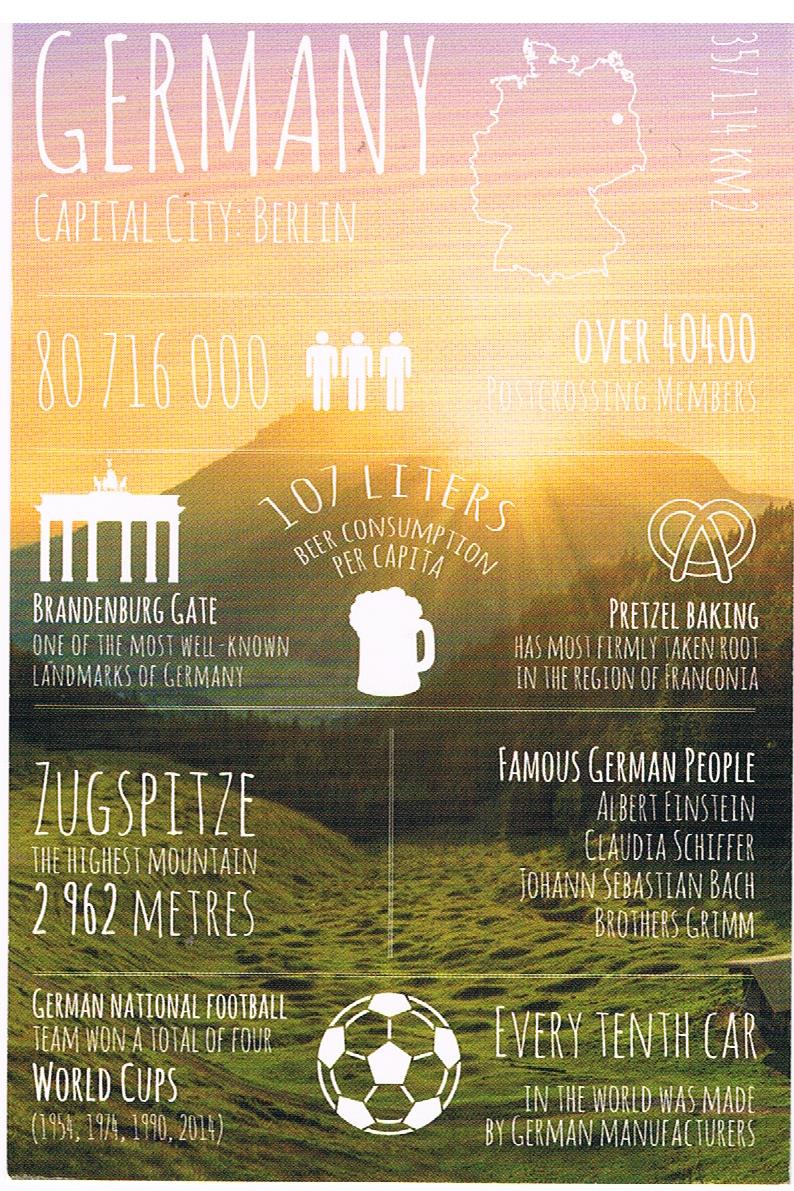The image depicts a picturesque landscape featuring a lush, grassy valley leading up to hills dotted with trees and culminating in a majestic mountain in the background. The sun is either rising or setting above the mountain, casting a brilliant array of orange and pink hues across the sky. The foreground and background together evoke a serene and vibrant natural scene. 

Overlaying this scenic backdrop is a detailed infographic about Germany. At the top left, the text reads "Germany, capital city Berlin," accompanied by a white outline map of Germany. Below this, it lists the country’s land area as 3,757,114 km². The infographic further details key statistics, including a population of 80,716,000, represented by icons of three human figures, and mentions "over 40,400 post-crossing members," although some of the text is partially obscured by the bright sunlight.

Incorporating both imagery and textual information, the infographic touches on prominent German cultural icons and facts, including:
- The Brandenburg Gate as one of the most well-known landmarks.
- Beer consumption averaging 107 liters per capita.
- The tradition of pretzel baking, particularly in the region of Franconia.
- The Zugspitz, Germany’s highest mountain, standing at 2,962 meters.

Additionally, it highlights famous German people such as Albert Einstein, Claudia Schiffer, Johann Sebastian Bach, and the Brothers Grimm. Another section celebrates the achievements of the German national football team, noting their four World Cup victories in 1954, 1974, 1990, and 2014. It also emphasizes Germany’s industrial prowess, stating that every tenth car in the world is manufactured by German companies. 

At the bottom, a soccer ball illustration reinforces Germany’s passion for football. The white text detailing these insights blends with the vibrant sky, occasionally making it challenging to read against the backdrop's intense colors.